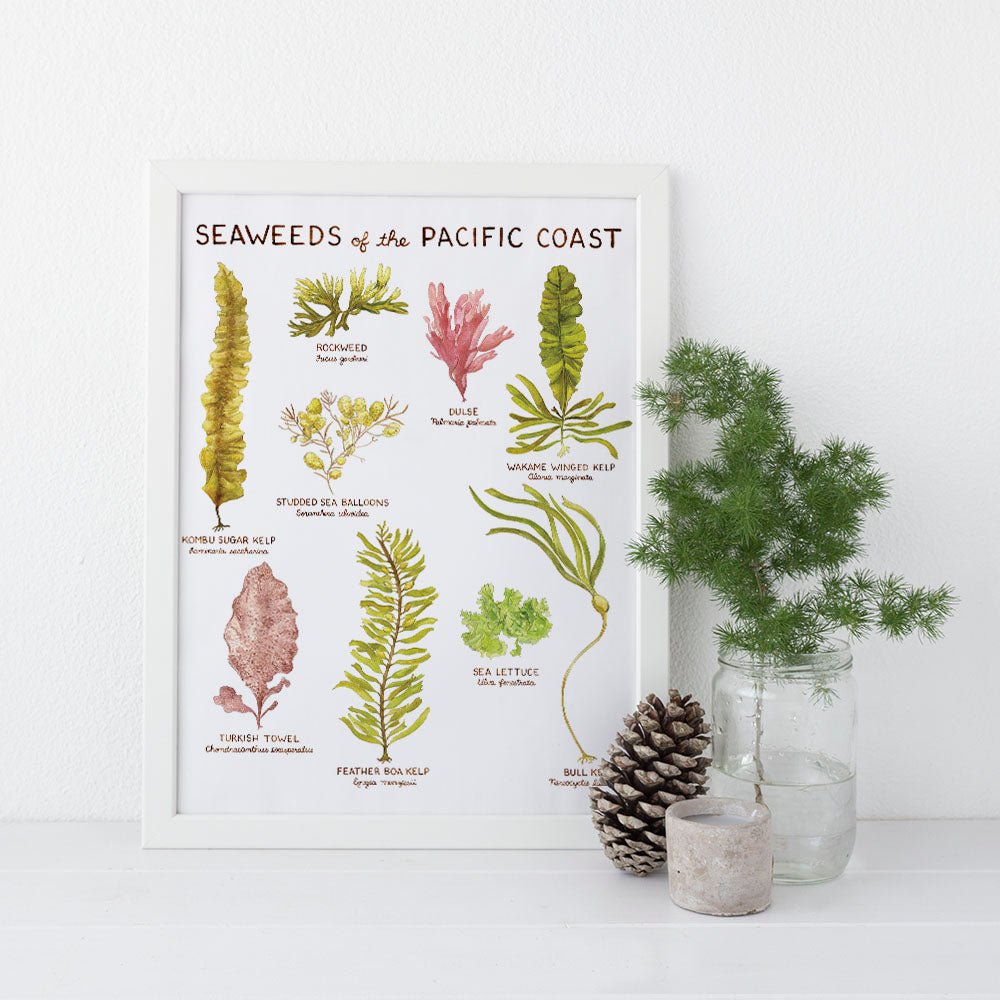In the image, a detailed chart titled "Seaweeds of the Pacific Coast" is prominently leaned against a white wall, nestled on a pristine white shelf. The chart showcases various types of seaweeds, each meticulously labeled, though the font is minimally legible. Noteworthy among these are rockweed, dulse, whack-em winged kelp, studded sea balloons, kombu sugar kelp, Turkish towel, feather boa kelp, sea lettuce, and bull kelp. The seaweeds are depicted in vivid colors, including shades of green, pink, and red, with some resembling floral arrangements and others displaying slender or broad leaves.

To the left on the shelf, a solitary pine cone stands subtly, its dark hue contrasting the white surroundings. Adjacent to the pine cone and slightly forward lies a small, circular candle. Near the candle, a mason jar half-filled with water supports a small, growing pine seedling, its vibrant green needles resembling those of a miniature Christmas tree. This scene is harmoniously set against the white shelf and wall, creating a serene and organized display.